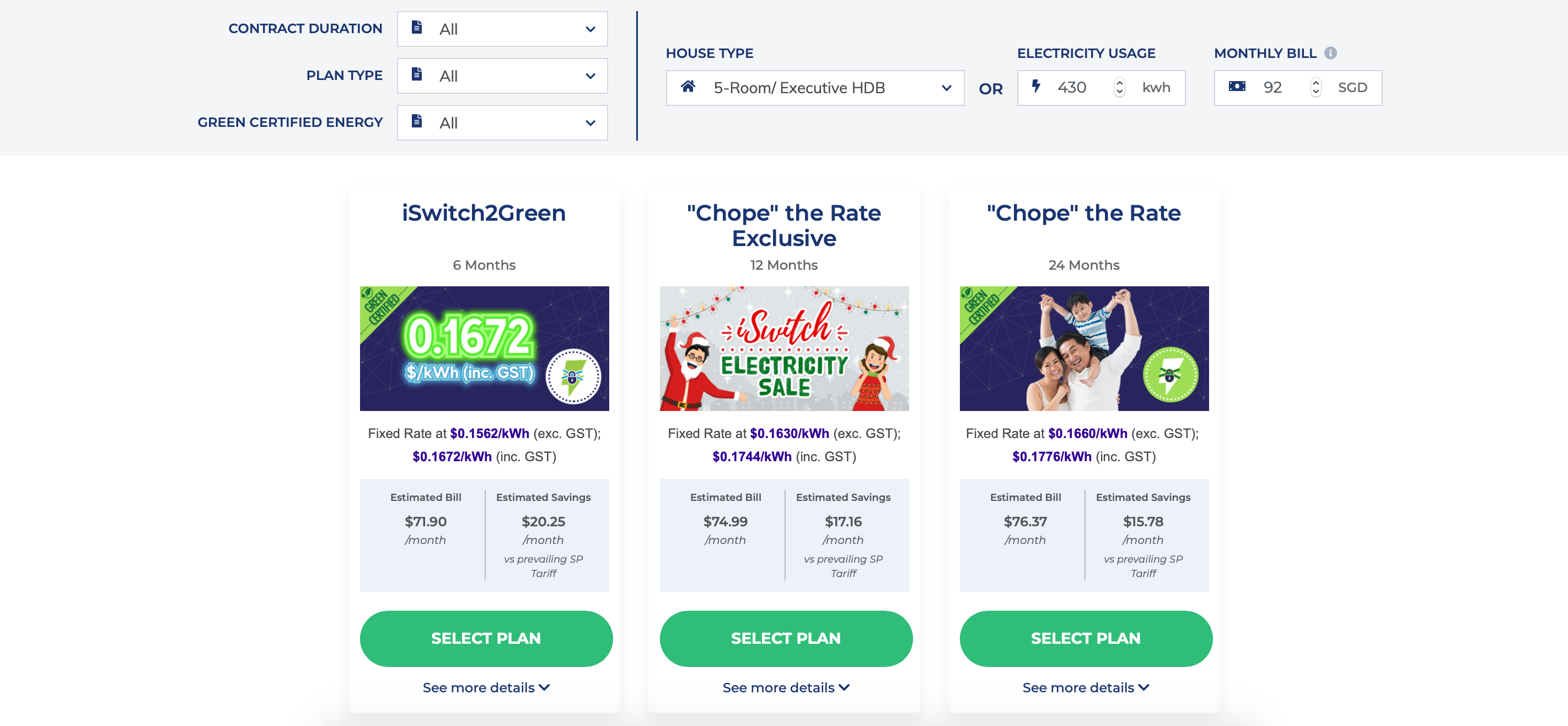This screen capture from a computer program displays an interface showcasing various electricity plans. The interface is divided into two main sections: a gray bar at the top housing several drop-down menus and a white background below featuring detailed plan options.

In the gray bar, users can filter their selections with the following options: 
- **Contract Duration**: Drop-down displays "All".
- **Plan Type**: Drop-down displays "All".
- **Green Certified Energy**: Drop-down displays "All".

To the right of these filters is a vertical separator line, followed by:
- **House Type**: Displayed as "5 Room Executive HDB".
- **OR**.

Below, the main heading reads "Electricity Usage" with a value of "430 kilowatt hours", adjacent to which the "Monthly Bill" is shown as "92 SGD".

The white background under the gray bar is split into three distinct plan options, each providing comprehensive data:

1. **Plan: I Switch to Green (6 months)**
   - **Cost per Kilowatt Hour**: 0.1672 SGD
   - **Fixed Rate**: 0.1562 SGD per kilowatt hour
   - **Estimated Bill**: 71.90 SGD per month
   - **Estimated Savings**: 20.25 SGD per month

2. **Plan: Chope the Rate Exclusive (Switch Electricity Sale)**
   - **Fixed Rate**: 0.1630 SGD per kilowatt hour
   - **Estimated Bill**: 74.99 SGD per month
   - **Estimated Savings**: 17.16 SGD per month

3. **Plan: Chope the Rate (24 months)**
   - **Fixed Rate**: 0.1660 SGD per kilowatt hour
   - **Variable Rate**: 0.1776 SGD per kilowatt hour
   - **Estimated Bill**: 76.37 SGD per month
   - **Estimated Savings**: 15.78 SGD per month

At the bottom of these three options, a unified "Select Plan" button is prominently displayed. The interface provides a clear, comparative overview of different electricity plans, aiding users in making an informed choice.